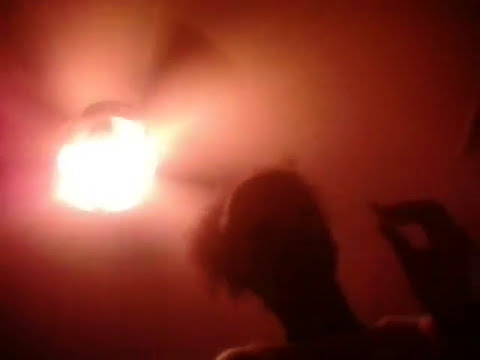The image features a young woman, possibly African-American, captured in a low-angle shot with a strong backlighting effect from a bright yellow ceiling fan light. This creates a striking yet shadowy atmosphere, bathing the room in a hazy red glow. The fan blades appear in silhouette, blurred by their motion. The woman's frizzy hair is pulled into a large bun, and she is positioned in the shadowy lower half of the image, making detailed features difficult to discern. She is gesturing with her left hand, although the specifics of her pose are lost in the shadows, adding to the overall mysterious and blurry quality of the photograph.